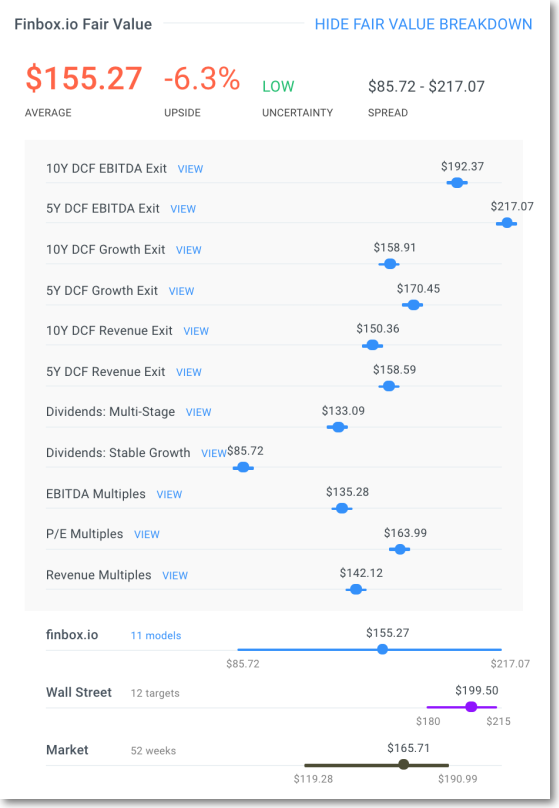Here is a detailed and cleaned-up caption based on the provided description:

---

The image is a screenshot featuring a prominent white box with a slight gray shadow along its right and bottom edges. Inside this box, various lines of text and numerical data are displayed. Starting from the top left, the text reads: "And then further to the right, it says," followed by another line of text below it in red which says, "In red text." Below this, in green text, appears the word "low." 

Continuing in black text, numeric values are shown: "$85.72 to $217.07," with the figures repeated as "$85 to $217.07." Further down, several headlines and data points are presented, accompanied by a chart featuring sliders.

The first line of data reads "$10Y DCF EBITDA EXIT VIEW $192.37," followed by a series of values:
- $217.07
- $158.91
- $170.45
- $150.36
- $158.59
- $133.09
- $85.72

Under the "EBITDA MULTIPLES VIEW" section, the following values are listed:
- $135.28
- $163.99
- $142.12
- $155.27
- $199.50
- $165.71

This detailed numerical breakdown appears to analyze financial metrics such as EBITDA exit views and multiples.

---